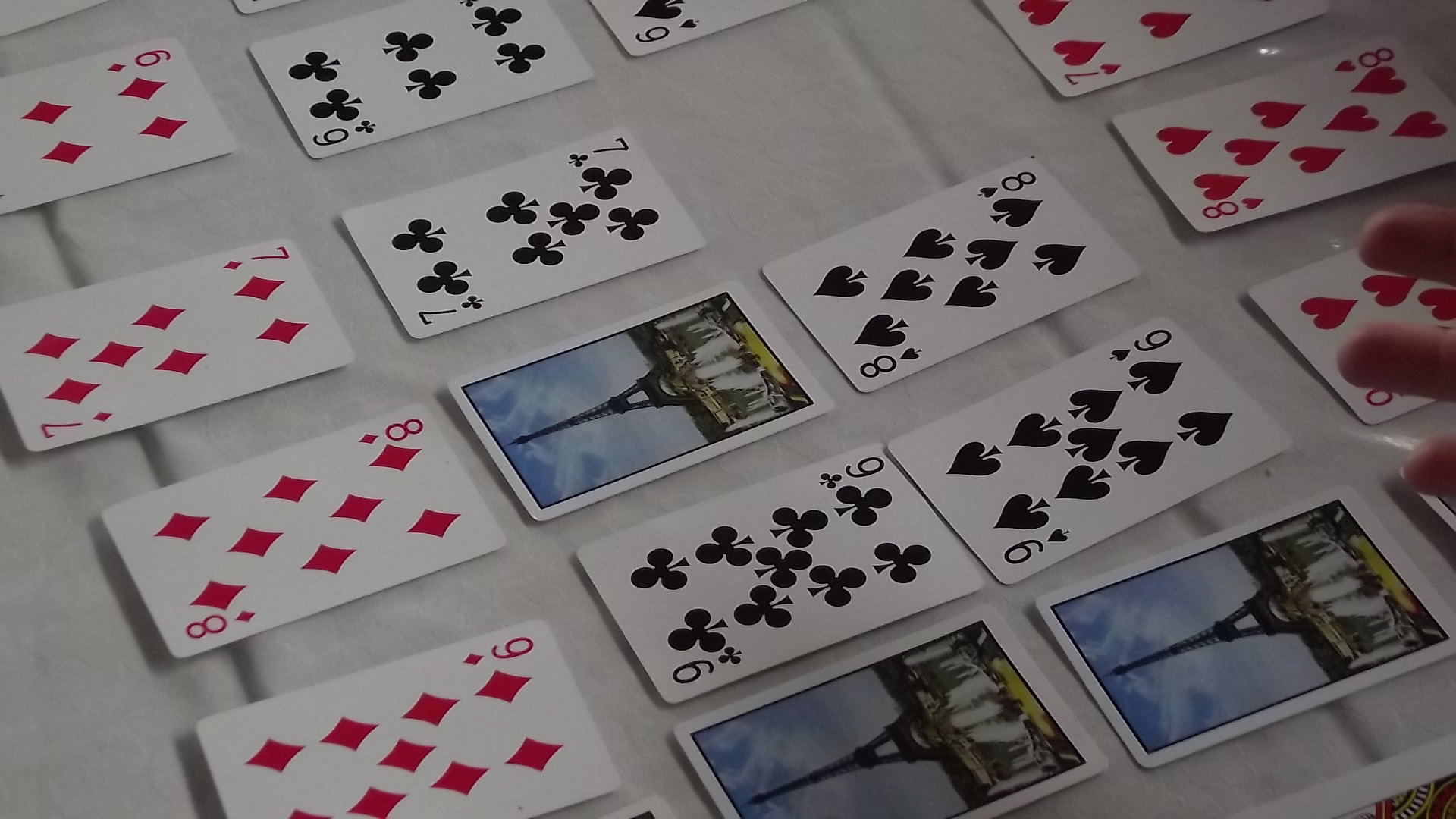The image features an array of playing cards meticulously laid out on a white tile table or counter. The cards are neatly organized by suit and in numerical order, prominently displaying the 6s, 7s, 8s, and 9s. A few cards are flipped over, concealing their faces but allowing for educated guesses about their identities. The reverse side of the cards showcases a design of the Eiffel Tower, set against a backdrop of blue sky with what appears to be a fountain in front of it.

On the far right edge of the photo, part of a person's hand is visible, specifically the index, middle, and ring fingers. The lighting in the image is somewhat dim, particularly on the right side, suggesting that the light source is closer to the left. The photo is captured at an angle, causing the rows of cards to lean to the left as they ascend. The obscured cards are likely the 8 of clubs, the 10 of clubs, and the 10 of spades.